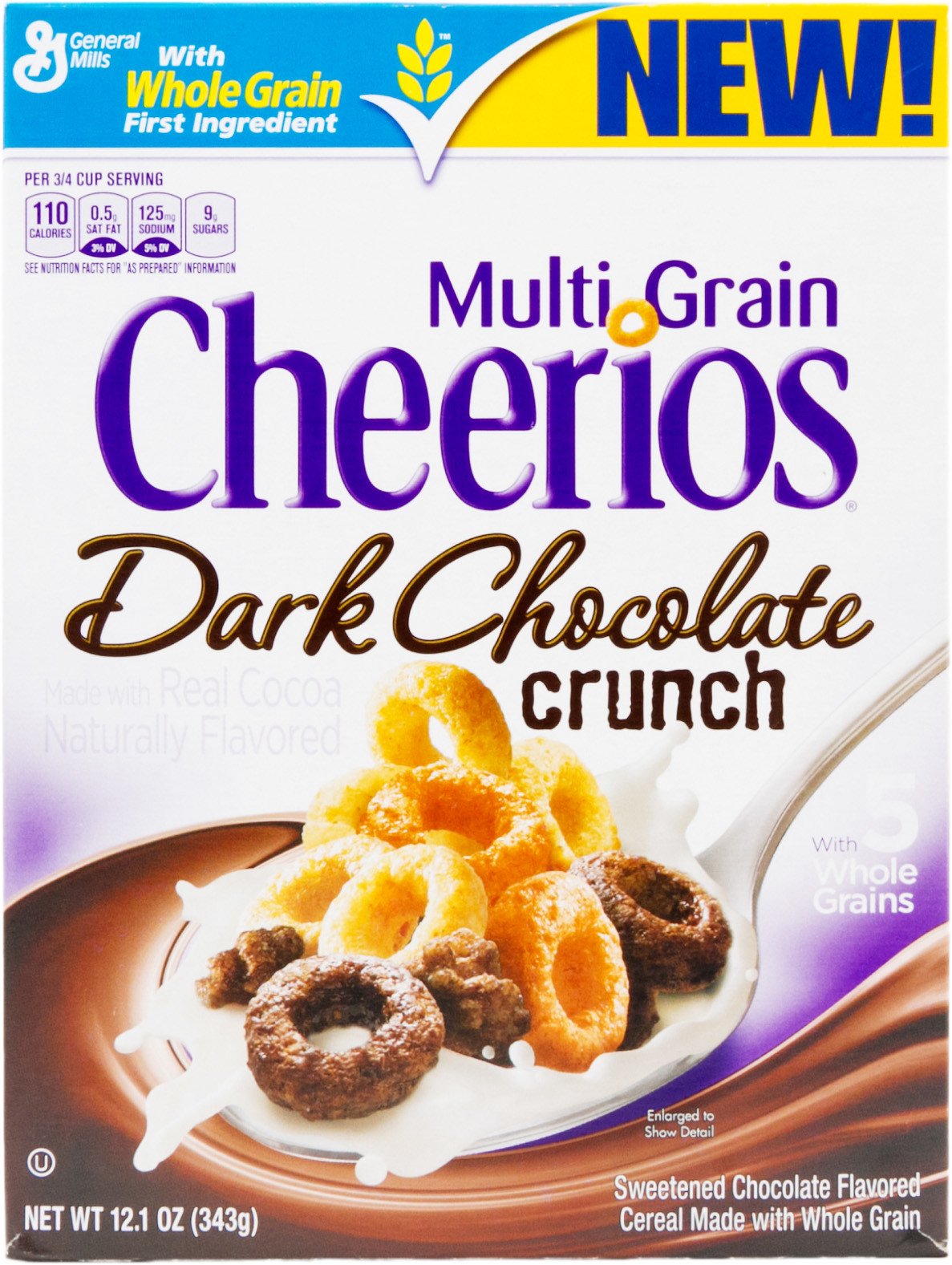Close-up of a General Mills cereal box featuring Multi-Grain Cheerios Dark Chocolate Crunch. The packaging highlights the fusion of multi-grain Cheerios and chocolate Cheerios with dark chocolate crunch pieces. A label on the front indicates that the cereal is sweetened and chocolate-flavored, made with five whole grains, emphasizing its healthy attributes. The top left corner presents nutritional information: 110 calories per three-quarter cup serving, likely excluding milk. The first listed ingredient is whole grain, underscoring the cereal's healthy positioning. The box features an eye-catching image of the cereal on a large spoon with milk splashes, accentuated by a prominent chocolate swirl, suggesting a decadent yet nutritious breakfast option. A disclaimer notes that the cereal image is enlarged to show detail, evoking a playful comparison to eating small doughnuts.